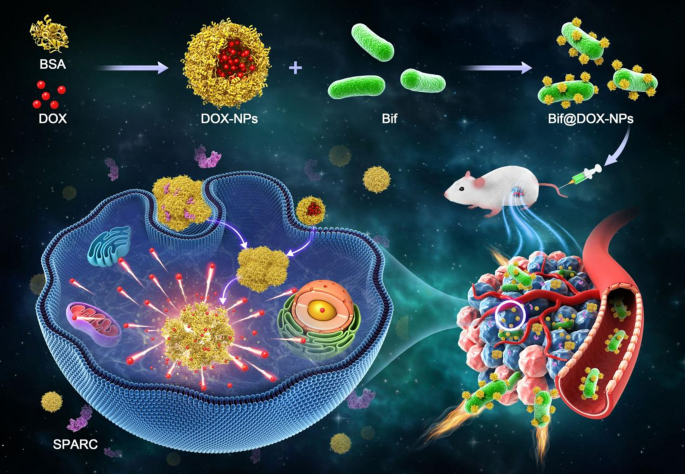This digital illustration, resembling a graph from a biology textbook against a dark, abstract background with green, cosmos-like patterns, meticulously maps a scientific process involving biochemical agents. At the top left, yellow strands labeled "PSA" and red dots labeled "DOX" combine to form "DOX-NPS," depicted as a circular structure with red circles. This combination is followed by the addition of "BIF," represented by green, bean-shaped bacteria. The merged entity, "BIF at DOX-NPS," is illustrated being injected into a mouse's tail. Inside the mouse, we see this composite flowing through its bloodstream, emphasizing how these elements interact within the organism. Finally, these components seem to enter a cell tagged "SPARC," culminating the biochemical journey depicted in this detailed illustration.